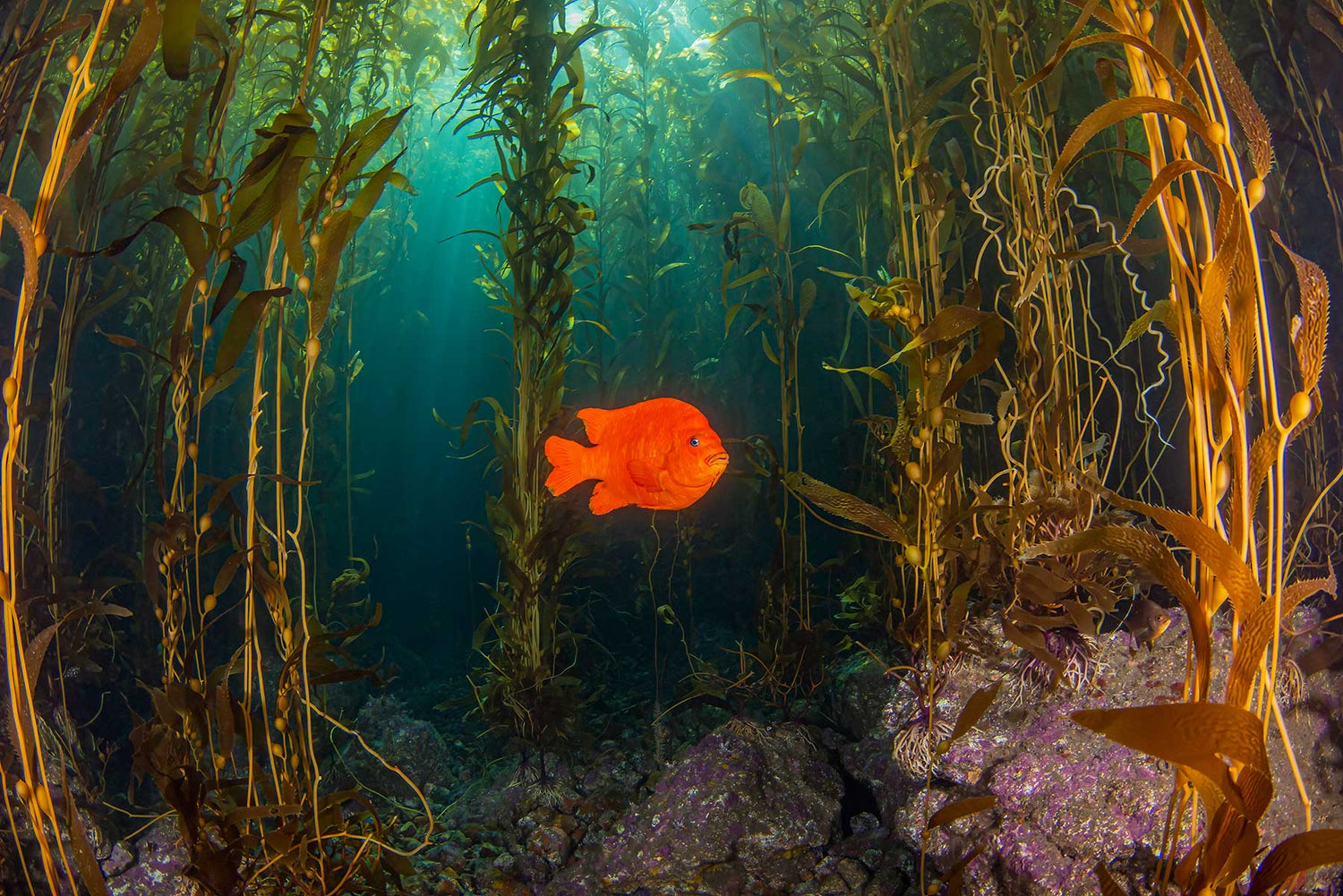This hyper-realistic image, whether it's an incredibly detailed painting or a professional photograph, captures the serene underwater scene of a single bright neon orange fish swimming alone. The fish, positioned prominently in the middle of the picture, draws immediate attention with one of its eyes clearly visible. Surrounding the fish are plants with leaves and algae that stretch vertically towards the lighter blue-green surface of the water, creating a network of yellowish-brown and green hues. The water's color gradient transitions to a darker blue towards the bottom. Below, the rough, rock formations and soil are depicted with complex textures featuring tones of brown mixed with purple and gray pigments. Illuminated by rays of light penetrating from the top, this underwater tableau is free of any text and exists in a pristine and tranquil aquatic environment, likely a pond, lake, or a secluded oceanic spot.